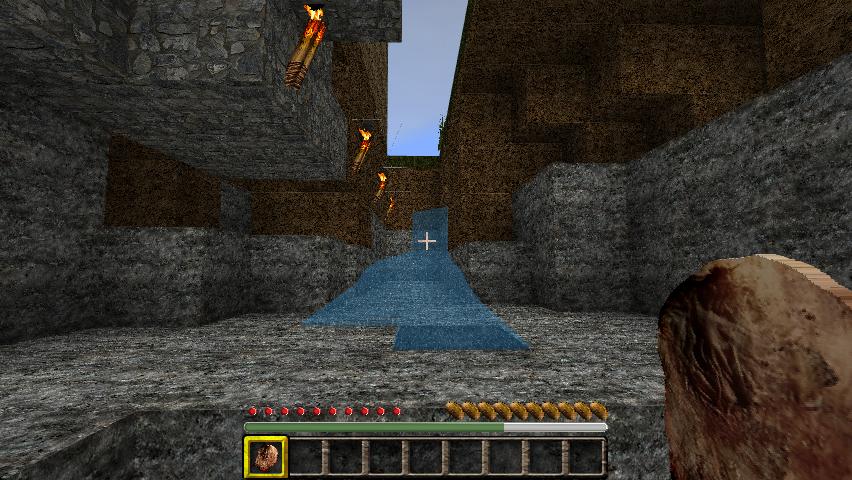The screenshot from a video game, displaying a first-person view reminiscent of Minecraft with potentially modded realistic textures, captures the player facing forward in a stone hallway or entryway. The scene is marked by gray and brown pixelated stone walls, with the blue shape and central tiny white cross suggesting a targeting reticle. Notably, there are a few flaming tiki torches affixed to the walls, casting a warm glow on the surroundings. At the bottom of the screen, there are several panels with black backgrounds and brown edges; the leftmost panel is highlighted in yellow, featuring a brown icon. Additional interface elements include a green progress bar, red dots, and brown icons. The player appears to be holding a brown, circular chip-like stone in their right hand, while water is visibly pouring in from above some dirt blocks directly ahead.